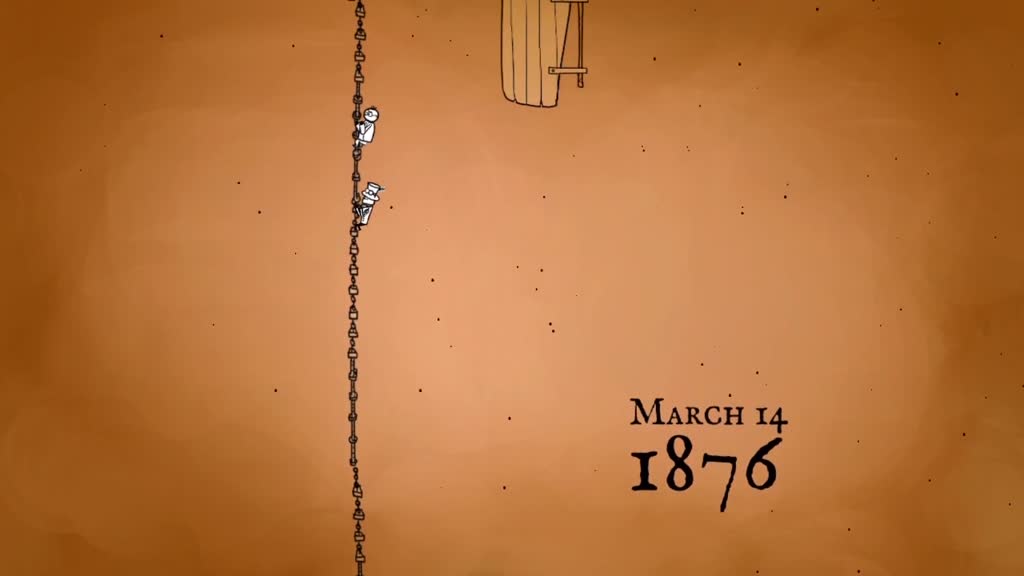This image features a hand-drawn cartoon illustration set against a predominantly light brown background with darker, almost circular shading around the edges, transitioning into some gray at the top. Black specks are scattered throughout the scene. Prominent in the center is a wooden scaffolding structure with a handle extending to the right, and on the left side, a chain or rope ladder extends vertically from top to bottom. Positioned about three-quarters up on this chain are two white stick figures, depicted as if they are climbing towards the top. The bottom right corner of the image is marked with the date "March 14, 1876" in black font.